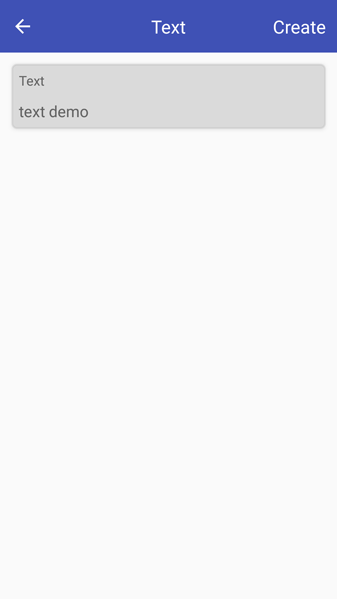This image appears to be a screenshot, possibly taken from a mobile application resembling the color scheme and design elements of Facebook. Dominating the top portion of the screenshot is a blue rectangular bar. On the far left side of this blue bar, there's a white arrow pointing to the left, indicating a back or return function. In the center of the bar, the word "TEXT" is prominently displayed in white capital letters. To the right side of this bar, the word "CREATE," also in white capital letters, is visible.

Below the blue bar, the background transitions to a clean white. Positioned centrally within this white space is a gray text message box. Inside this gray box, the word "TEXT" appears, followed by the phrase "text demo" on the subsequent line. The overall layout suggests this could be a user interface for entering or reviewing text messages, with a clear and minimalist design that focuses on functionality and readability.